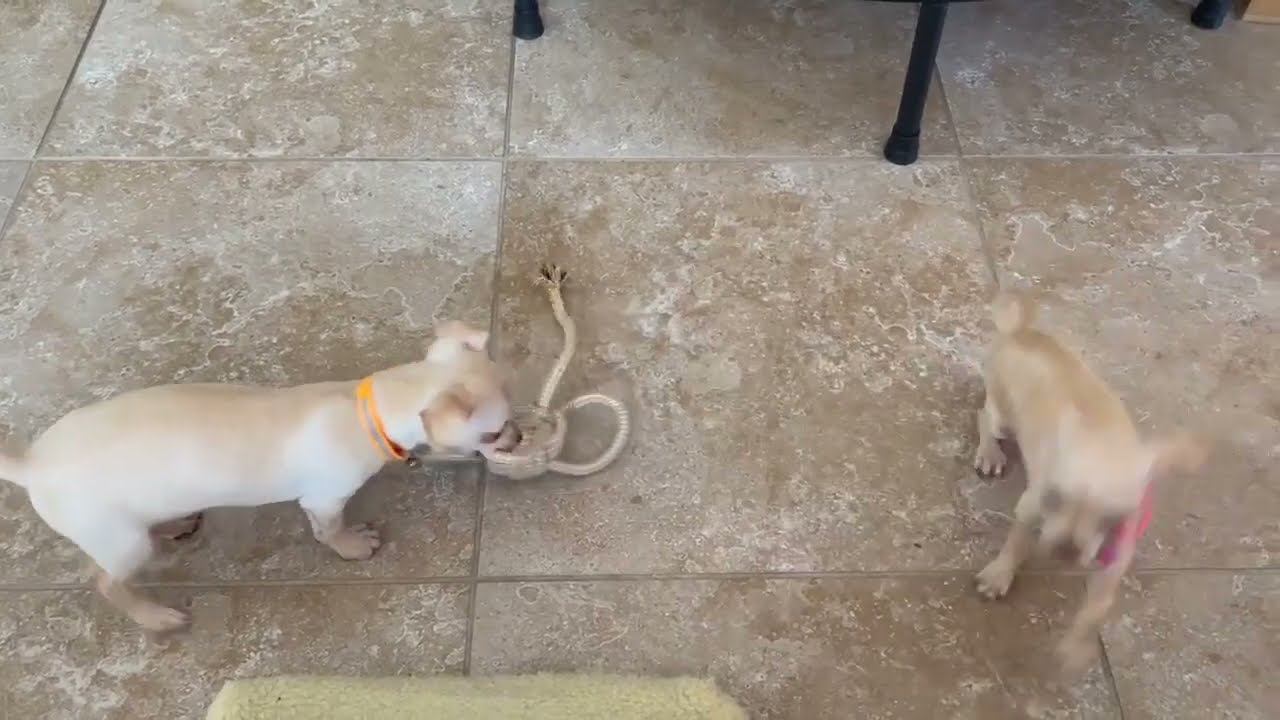The image captures an energetic scene with two young, light brown puppies playing on a patterned, stone-tiled floor, which features a mix of light and dark tan colors with white stains. The puppy on the left, with an orange collar, is standing sideways to the camera and engrossed in playing with a chew toy that has a rope extending from it. Meanwhile, the puppy on the right, a bit blurry due to its motion, appears to be mid-jump, exuding a sense of excitement. It has a pink leash visible on the left side of its head, hinting at its playful nature. The legs of a chair extend into the top of the image, and a yellow rock can be seen partially at the bottom, adding to the playful setting of the scene.